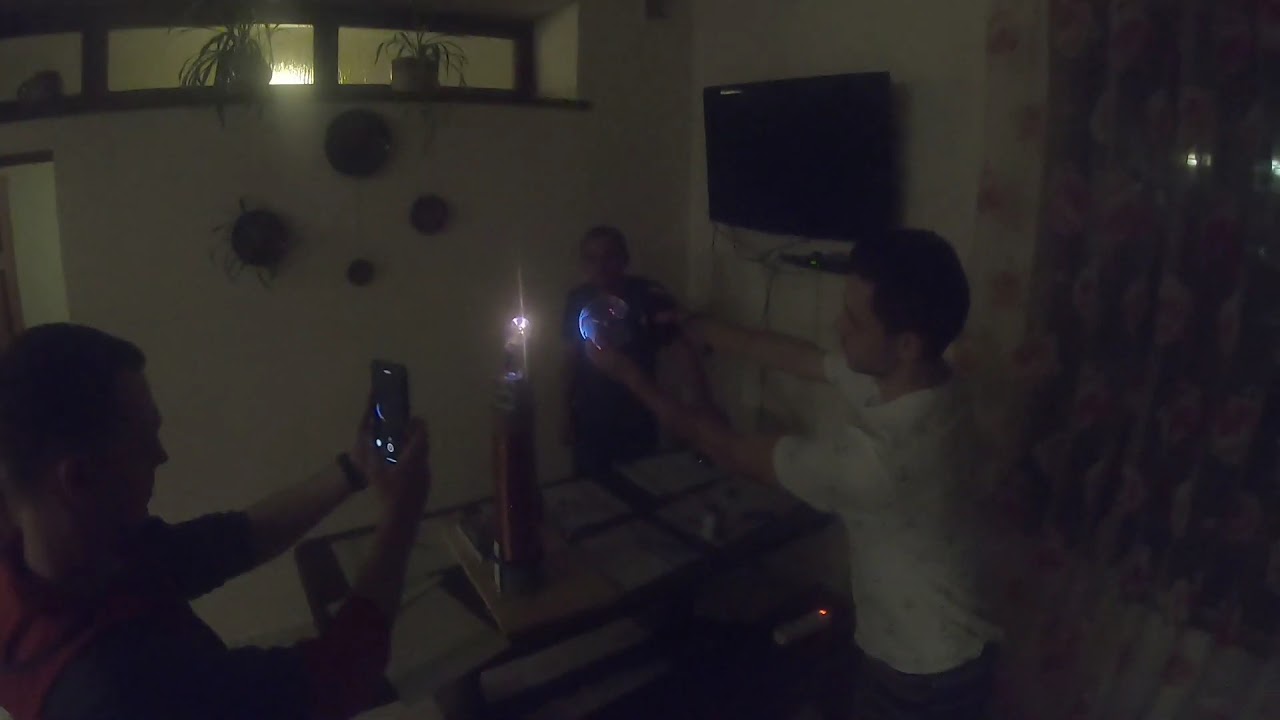The image depicts a dimly lit room with three people inside, gathered around a table. At the center of the table is a tall, thin, cylindrical object with a light on top, which seems to be the focal point of their attention. The room ambiance suggests either a living room or dining room setting.

One man in the foreground is holding what appears to be a camera phone with both hands. He is wearing a red sweatshirt and has short, dark hair. To his right stands another man in a white shirt, also with short, dark hair. He appears to be holding a small, possibly reflective spherical object, which might be a crystal or disco ball. In the shadows to the back, there is a third person, partially obscured and wearing glasses.

Decorating the room is a TV mounted on the wall to the right, which is turned off. High on the left wall, small windows feature potted plants on their sills. Additional decorations include three blurry circular objects, possibly plates, hanging on the wall. The lighting is minimal, adding to the overall dark and grainy quality of the photograph.